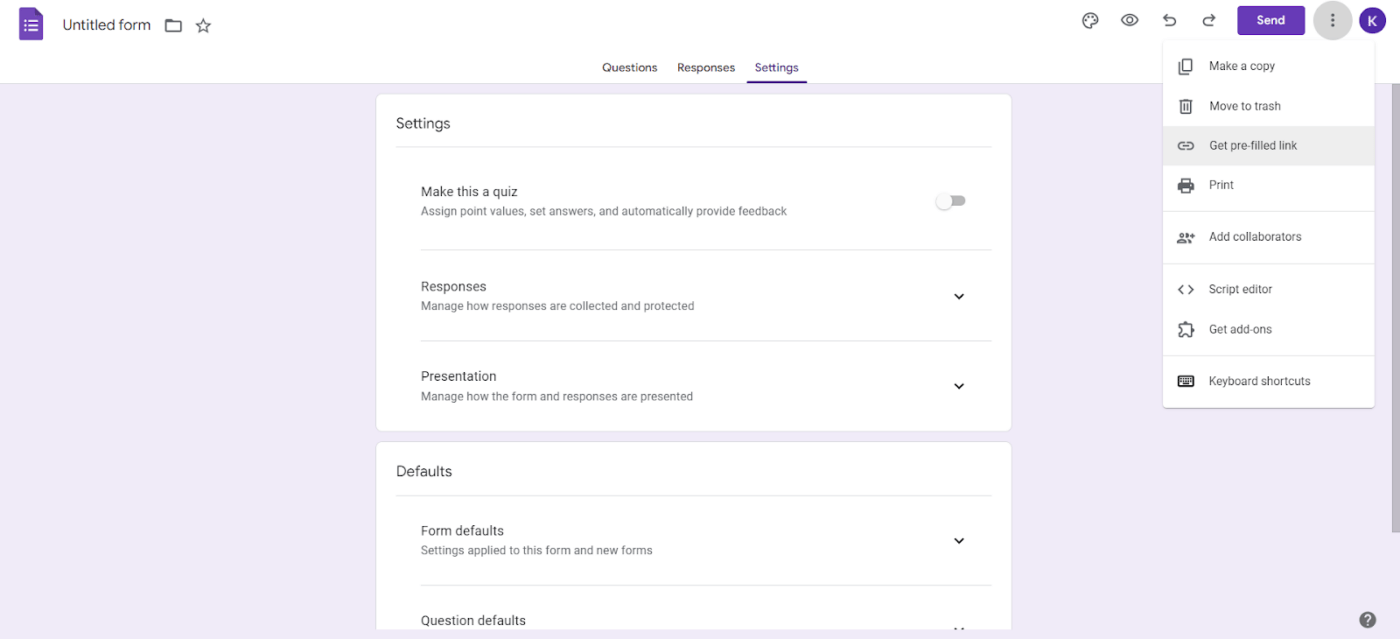The image displays a Google Form interface. In the upper-left corner, there is an "Untitled form" label accompanied by a small purple page icon with white lettering. To the right, the file options are visible, including "File," "Favorite," and further to the right, there are three main tabs: "Questions," "Responses," and "Settings." The "Settings" tab is currently selected, indicated by an underline and purple color.

In the "Settings" section, several options are listed:

- **Make this a quiz:** Allows users to assign point values, set correct answers, and provide automatic feedback. A toggle button is available to enable or disable this feature.
- **Responses:** Manage the collection and protection of responses with a drop-down menu.
- **Presentation:** Control how the form and responses are displayed using a drop-down menu.
- **Defaults:** Deals with the form and question defaults. Any changes here apply to the current form and new forms subsequently created.

On the upper-right side, there are several icons including a palette (theme customization), an eye (preview), arrows (navigation), and a purple "Send" button with white text. A context menu, denoted with a triple-dot icon, is currently expanded and highlighted in gray. It provides various options: "Make a copy," "Move to trash," "Get pre-filled link," "Print," "Add collaborators," "Script editor," "Get add-ons," and "Keyboard shortcuts."

To the top-right, there's a purple circle containing a white "K," possibly representing the user's profile. In the bottom-right corner, a question mark icon offers help resources. The background color of the interface is a light grayish-purple, and the settings menus and boxes are white with black text.